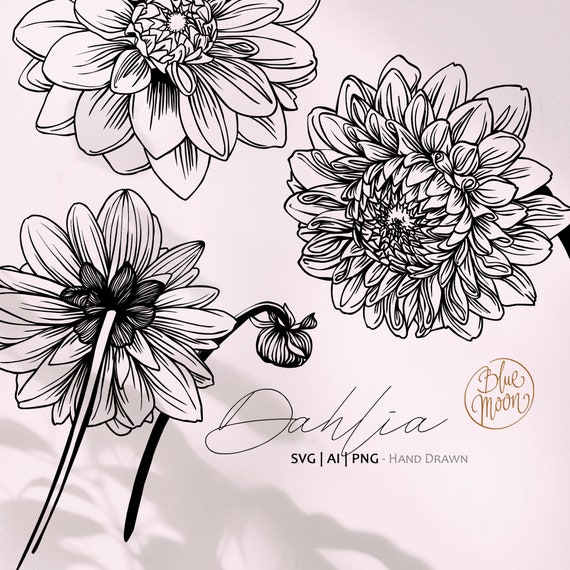The hand-drawn image features a collection of flowers positioned across a subtle gray background with a hint of light wine color. On the right side, there are two flowers: the top one is fully facing forward, while the one beneath it leans to the left. On the bottom left of the image, there's the back view of another flower next to a closed flower bud. Below these, the word "Dahlia" is written in thin cursive script, followed by the typescript "SVG | AI | PNG" with the notation "hand-drawn" nearby. Above this text, a circle contains the phrase "Blue Moon" in a slightly different script style. The drawing captures various stages of the flowers' growth, with one still in bud form and others in varying degrees of bloom, each detailed with multiple petals and stems subtly shaded in the background.